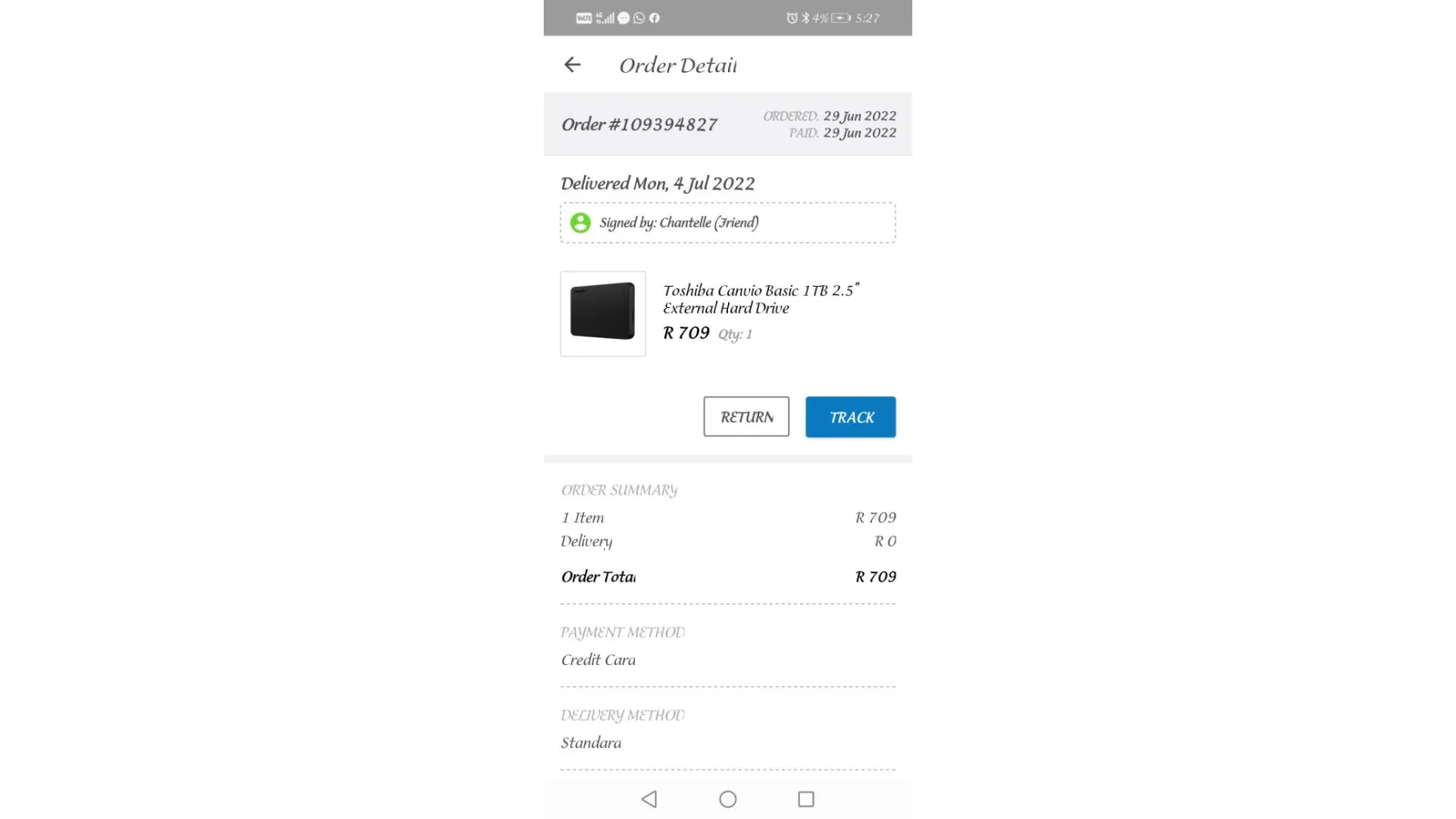The image shows a smartphone screen displaying detailed order information. At the top of the screen, within a gray bar, the phone's battery life and the time, 5:27, are visible. Below this, there is a white section with a left-pointing arrow labeled "Order Details." Further down, a gray area details the order number, "109-394-827," and specifies the order and payment dates as 29 June 2022. 

The following white section highlights the delivery status, reading in black text: "Delivered Monday, 4 July 2022, signed by Chantel (friend)." Adjacent to this text is an image of a black box. Next to the image, the product information lists: "Toshiba Canvio Basic 1T, external hard drive," along with the price, "R709," and quantity, "1."

Below that, two buttons are displayed: a white "Return" button and a blue "Track" button. Beneath the buttons, an "Order Summary" section notes: "1 item, R709, delivery R0, order total R709."

Finally, towards the bottom of the screen, the "Payment Method" is specified as "Credit Card," and the "Delivery Method" is labeled as "Standard."